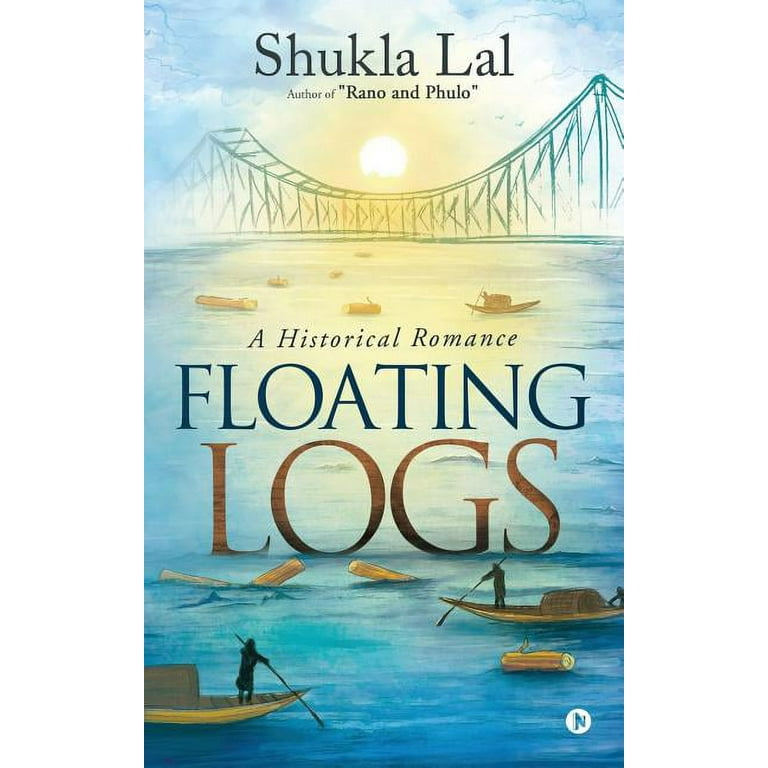The book cover illustration features a serene ocean scene with shades of blue, beige-ish tan, brown, gray, black, and white. In the foreground, several small pontoon boats float on the water, each occupied by people rowing with oars. Scattered among the boats are floating logs. Dominating the background is a large, impressive bridge with the sun rising or setting behind it, casting a yellow and white glow. The artwork appears to be rendered in watercolor and color pencil, adding a soft, dreamy quality to the image. At the top of the cover, the title reads “Floating Logs” and the author is Shukla Lal. The cover also mentions that it is a "Historical Romance."